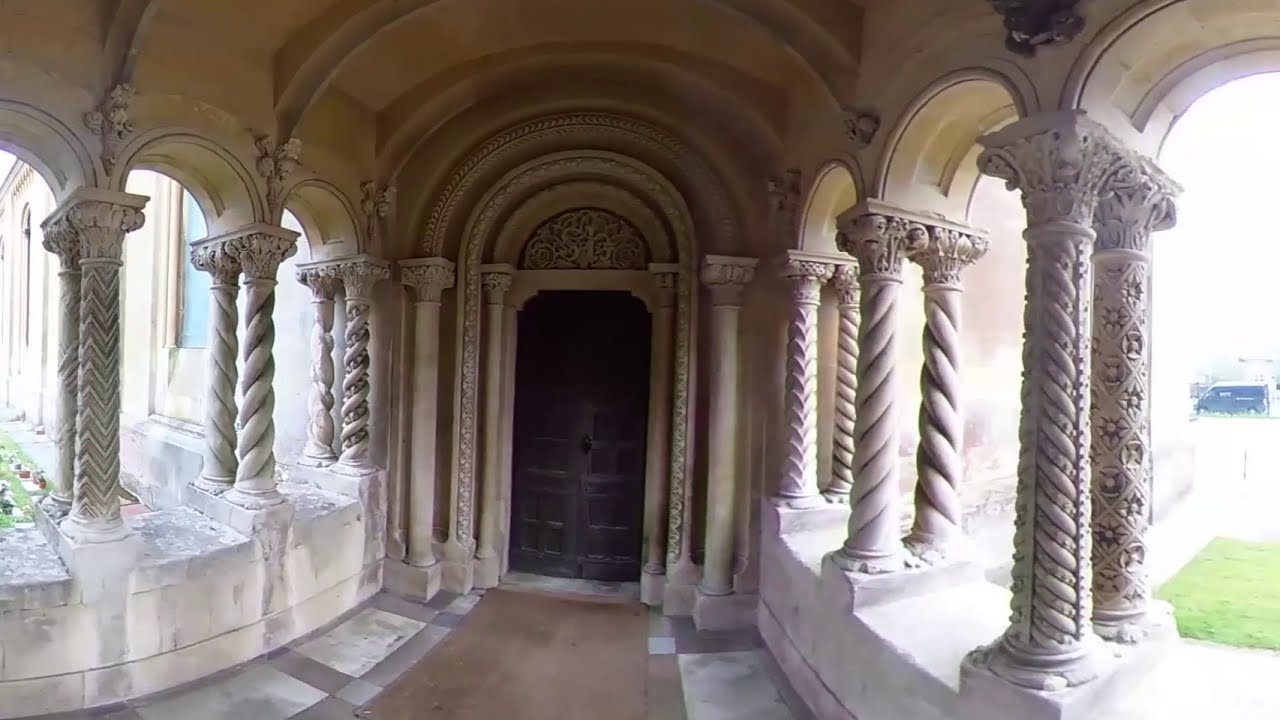The image depicts the grand entrance to a building reminiscent of an Italian cathedral or a Greek palace. The structure boasts large, ornate columns that support an arched roof, with intricate, unique designs adorning each column. The building's façade is a white-beige hue, heightening its classical, stately appearance. A beautifully crafted, heavy brown door, shaped like an archway, sits prominently at the entrance, with an ornate feature crowning it. 

The walkway leading to the door is flanked by light brown paths and cement borders. To the left, a lush garden with green grass and windows with arched tops enhances the serene outdoor ambiance. In the background, an area, possibly a yard, stretches out with more green grass, and a vehicle that appears to be an Amazon Prime van, either black or blue, is parked by the street. The scene combines the elegance of historical architecture with subtle modern elements, creating a visually striking composition.